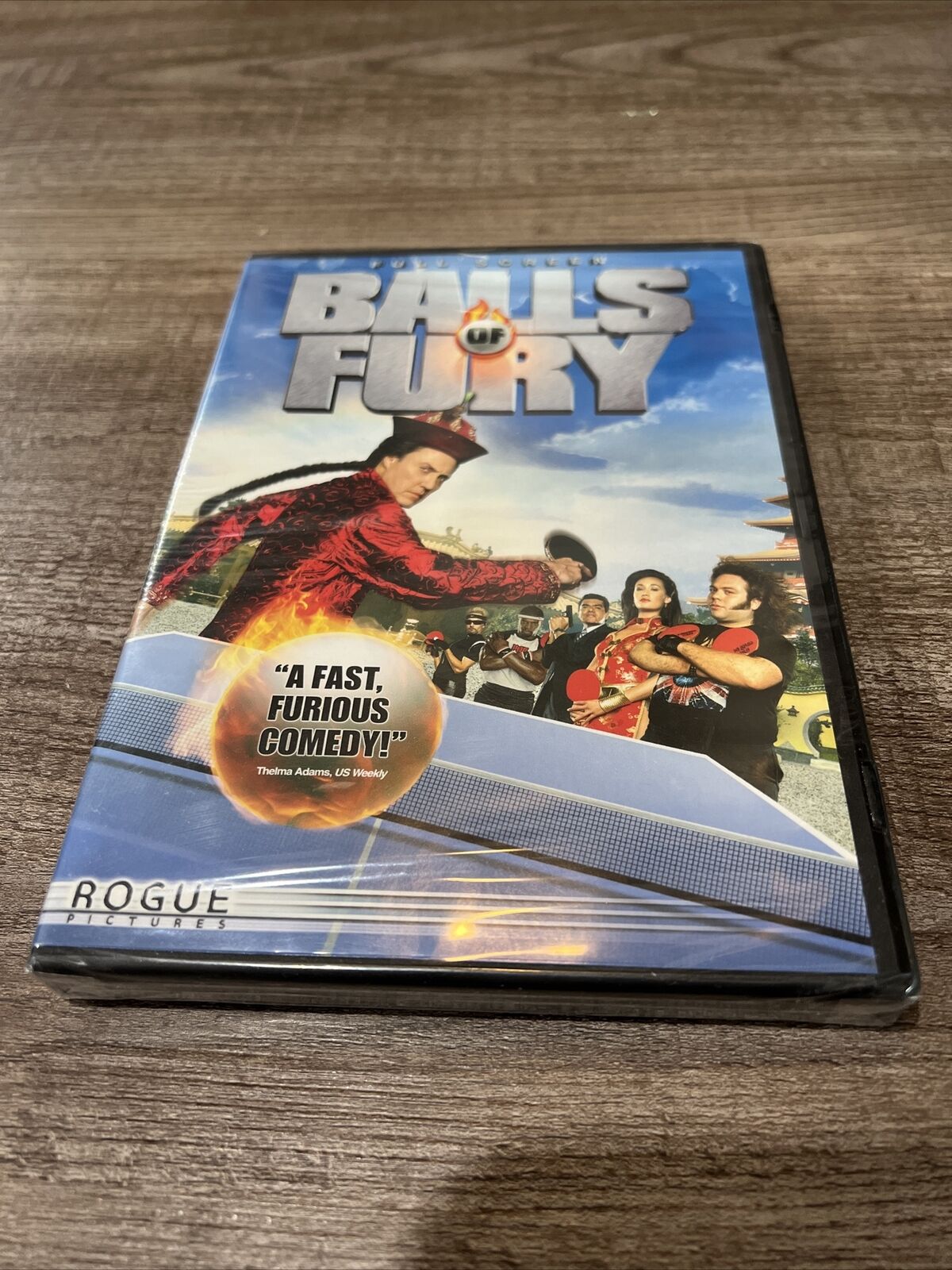The image showcases a DVD case of the movie "Balls of Fury" lying on a dark gray wooden floor. The title "BALLS OF FURY" is prominently displayed in gray, all-capital font at the top of the front cover. The cover features multiple characters from the movie, centralizing a man wearing a traditional Chinese red robe, possibly a kimono, in an action pose hitting a ping pong ball. Surrounding him are additional characters, including a woman also dressed in red Asian attire, and several men wearing various outfits such as a suit and t-shirts. A blue box occupies the bottom part of the case, which includes a yellow circle with the quote "A Fast Furious Comedy." In the bottom left corner, the text "Rogue" indicates the production company. Overall, the image vividly captures the lively and action-packed essence of this ping pong-themed comedy film.